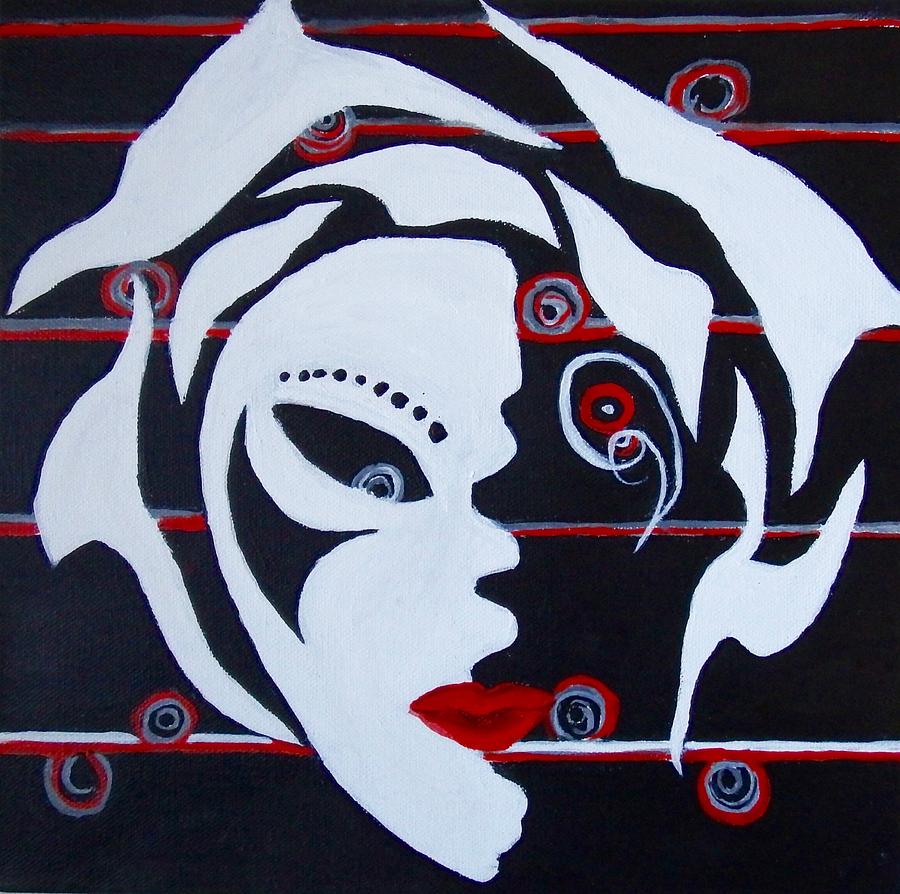This detailed abstract painting presents a striking modern depiction of half a face set against a dark, complex background. The background is primarily a deep dark blue interspersed with red and lighter blue lines, resembling crashing waves dotted with small circles in alternating colors. Stripes of red and gray run across the composition at regular intervals. These stripes are punctuated with patterned circles featuring concentric rings of black, gray, red, and white, creating a rhythmic and layered texture.

The focal point of the painting is a meticulously detailed half-face. The right half of the face is rendered in stark white, with piercing blue eyes and eyebrows. The contrasting left half merges seamlessly with the dark, intricate background, where the eye appears as a small red circle with a white dot at its center, enhancing the abstract nature of the piece. This eye is surrounded by spirals and dot patterns, introducing a sense of depth and movement. Noteworthy features of the face include bright red, vividly defined lips and an exaggeratedly long and pointy chin, adding a surreal dimension to the figure. The white depiction of hair on the face emphasizes the graphic quality of the portrait.

Overall, this artwork merges diverse graphical elements and abstract shapes to create a visually captivating and rich portrayal of half a face amidst a dynamic, colorful background.